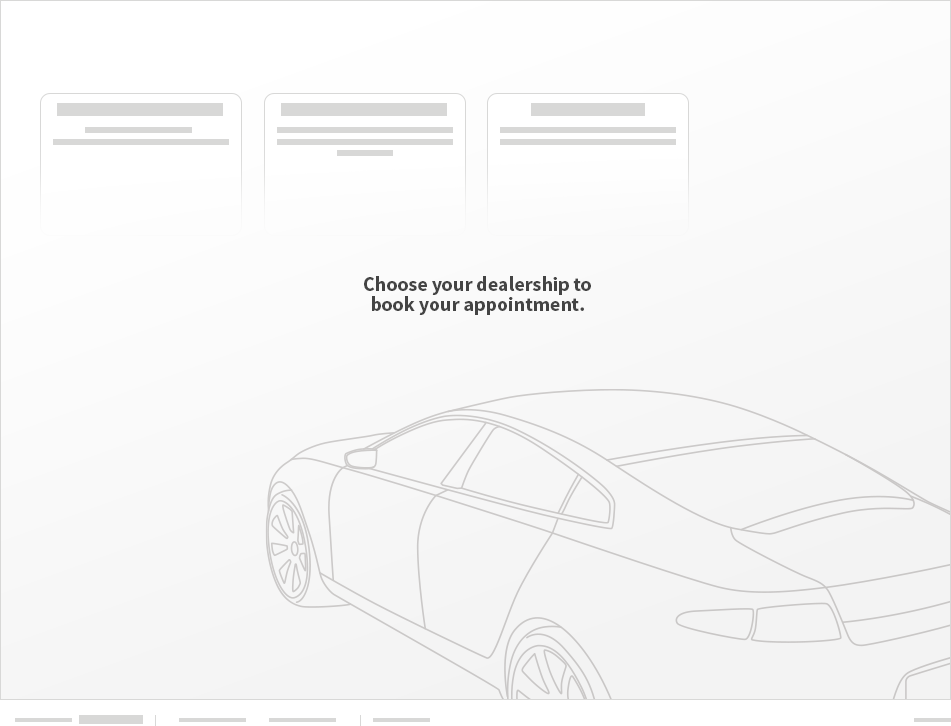This image is a monochromatic, black and white design resembling a website template for a car dealership. The primary visual element is the distinct outline of a car, sketched in gray lines, positioned such that its rear and left side are visible, facing the top left corner. The vehicle showcases an elegant, curvaceous profile, suggesting a sporty, luxurious four-door model with large rims and thin tires.

At the center of the image, bold black text reads, "Choose your dealership to book your appointment." Directly above this, three partial squares (each missing one side) are aligned horizontally, containing grey horizontal bars of varying numbers—three bars in the first square, four in the second, and three in the third. These elements likely indicate placeholders for additional information.

The background is a clean white, providing contrast to the design elements, and additional faint gray bars are visible toward the bottom edges of the image, enhancing the structured aesthetic indicative of a dealership advertisement.